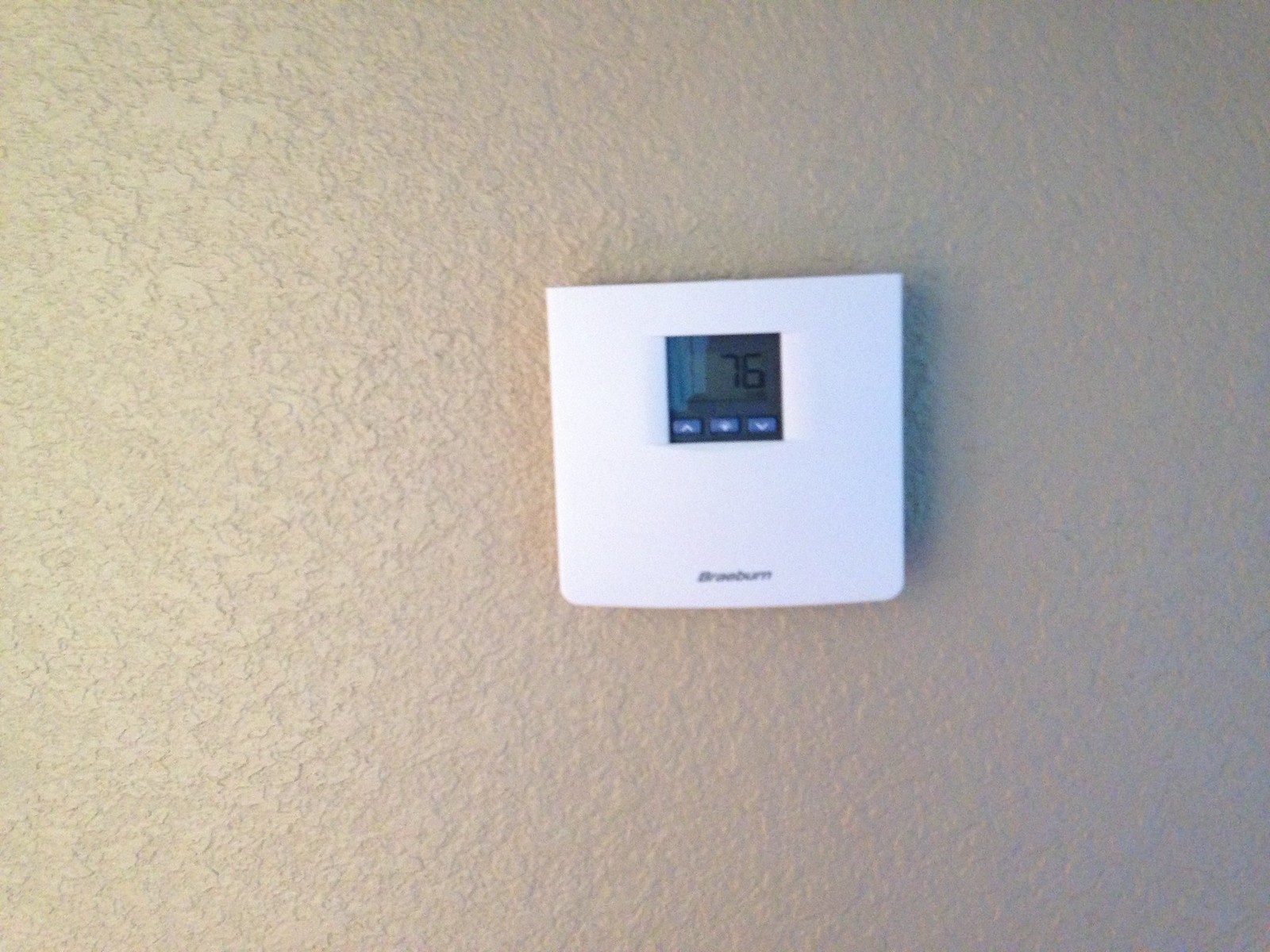The photograph captures a temperature controller mounted on a plaster-finished wall with a rough texture and cream color. The temperature controller, constructed of bright white plastic, stands in stark contrast to the wall. It has an oblong shape, featuring the manufacturer's name in black at the bottom, though the letters are partially obscured. Dominating the center of the device is a small digital screen, approximately 1 inch by 1 inch, which displays the faint number "76" in black against a grey background. Beneath the screen are three small buttons in blue, marked with white indicators: an up arrow, an off symbol, and a down arrow. The photograph is slightly shadowed on the left side, adding depth to the scene.